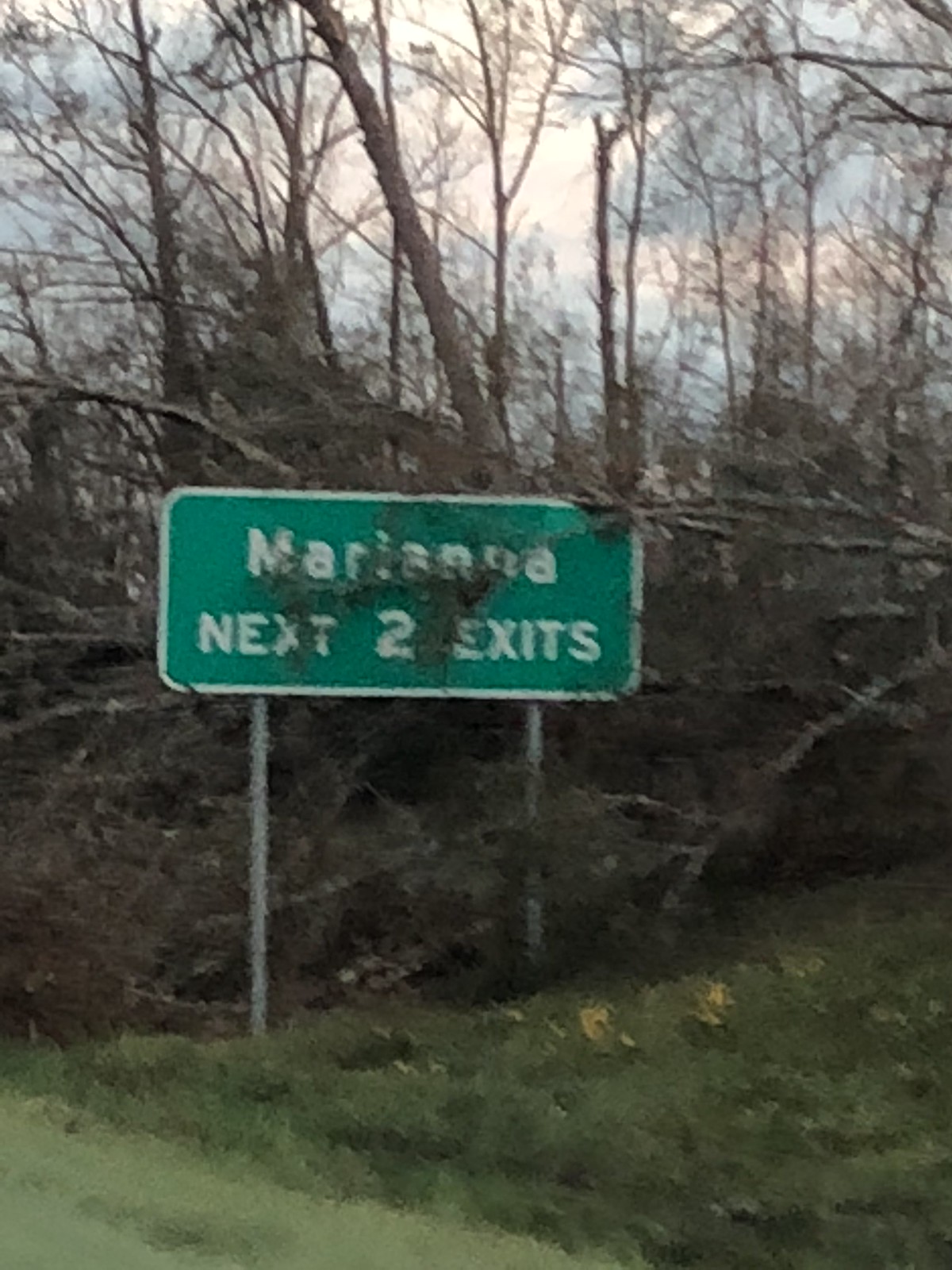This photograph captures a scene along the side of a highway as viewed from a moving vehicle. Central to the image is an oblong, rectangular highway sign outlined in white and featuring a green background with white lettering. The sign reads "Mariana" in capital letters at the top and "Next Exit" directly below it. It's mounted on two sturdy silver steel poles.

Surrounding the sign is a dense backdrop of woods, where several trees appear to have fallen, with one large branch noticeably draped across the sign. The ground in the foreground is covered with a patch of green grass, leading up to the sign. In the background, the sky is a bright blue, adorned with a few wispy white clouds, adding a serene touch to the scene. The juxtaposition of nature's quiet beauty and the man-made structure creates a striking visual contrast.